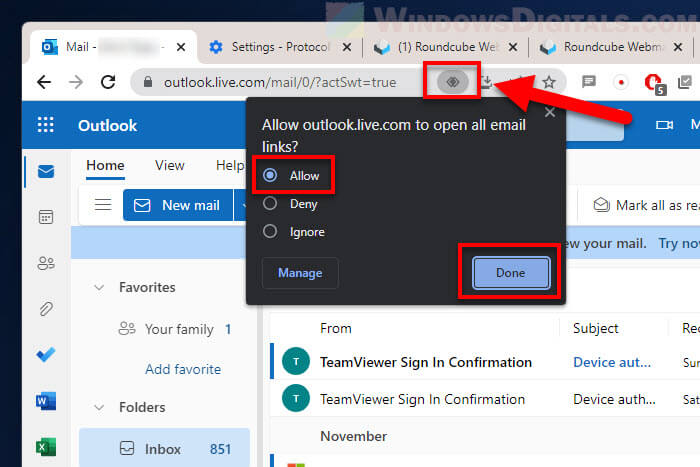Screenshot of a Microsoft Outlook training session. The Outlook interface displays various emails and folders on the left-hand side, typical of the email client layout. In the center of the screen, a prominent black pop-up box is overlaid, containing options and instructions for using one of Outlook's search features. The pop-up box highlights a specific button on the Outlook search bar that enables Outlook Live to open and search through email links. Additionally, the "Done" button is also emphasized, indicating the completion of the task. This training content, sourced from WindowsDigital.com, aims to guide users through effectively utilizing this particular feature of Microsoft Outlook.